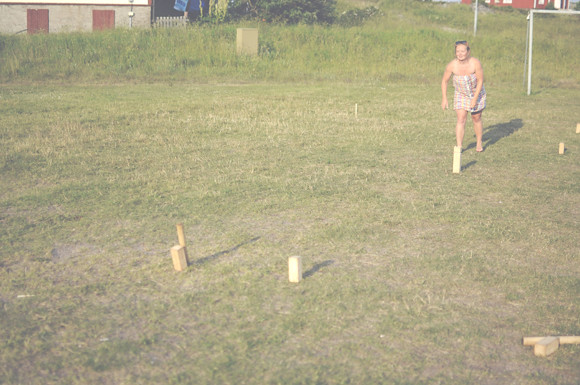The image depicts a tanned Caucasian woman standing barefoot on a grassy field, the ground showing patches of brown amidst the sparse green, suggesting the need for water. She is intently focused on a game involving short, rectangular wooden blocks and small wooden poles, one of which she appears to have just thrown. She is dressed in a sleeveless, halter-type dress that reaches her knees, with shorts peeking underneath, and she has sunglasses resting on top of her head. In the background, there is a soccer goal stand, although she is not engaged in soccer, as well as various structures: a beige building with red doors, another red building with white doors, and tall green shrubs. The scene captures her amidst this curious game that resembles a combination of lawn bowling and ring toss, her shadow stretching behind her in the outdoor light.